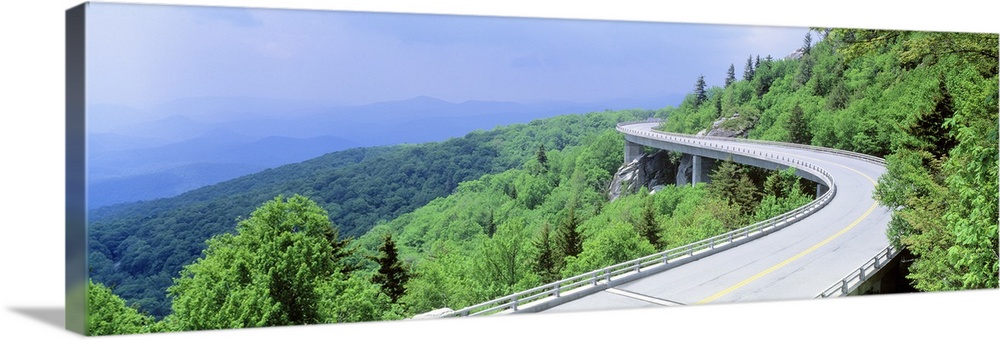This image is a detailed digital mock-up of a beautiful outdoor landscape, portrayed on a wide, raised canvas print. The scenic view prominently features an elevated, curving two-lane highway that winds around a densely forested hillside, supported by concrete pillars. The road, marked by a yellow dividing line and guarded by metal railings on both sides, creates an S-shaped path as it navigates the mountainous terrain. On the right-hand side of the image, lush green trees blanket the hillside, cascading downwards into a valley. The left side of the elevated road is fringed with brighter green treetops, transitioning to darker shades as they recede into the background. In the distance, layers of rolling hills and blue mountains are visible, blending seamlessly into a sky that fades from light to darker blue. The canvas itself adds depth to the landscape, enhancing the three-dimensional effect of this picturesque scene.